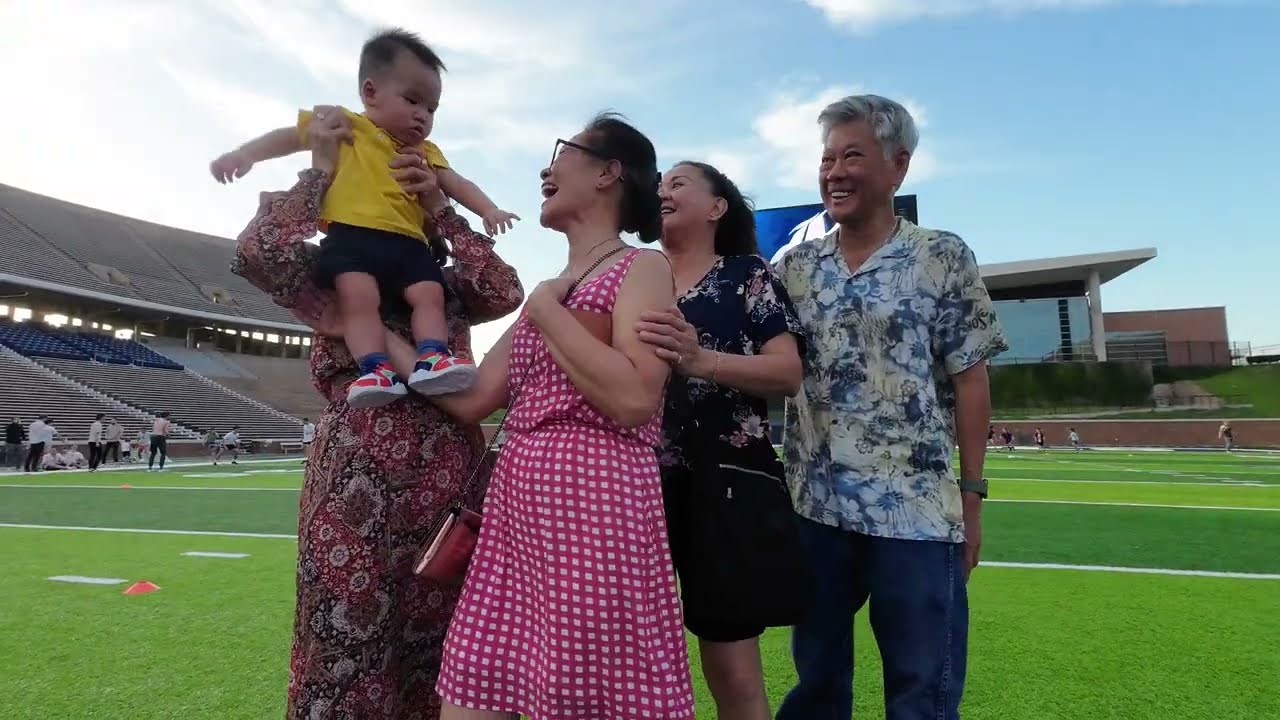A family of five, appearing to be of Asian or Pacific Islander descent, stands together on a vibrant green football field with stadium bleachers visible in the background. They are gathered in a semicircle, all facing towards the left side of the image and smiling at a baby. The baby, who is held up in front of a woman's face, wears a yellow shirt, blue or black shorts, blue socks, and red and white shoes. The woman holding the baby is dressed in a dark outfit. Next to her is an older woman with glasses, her hair in a bun, donning a red and white checkered dress and a shoulder purse. Beside her stands another woman in a dark shirt with floral patterns and a dark skirt. On the far right, a man smiles warmly, dressed in a light cream and blue or green floral Hawaiian shirt. They all look happy and are enjoying a joyful moment together.